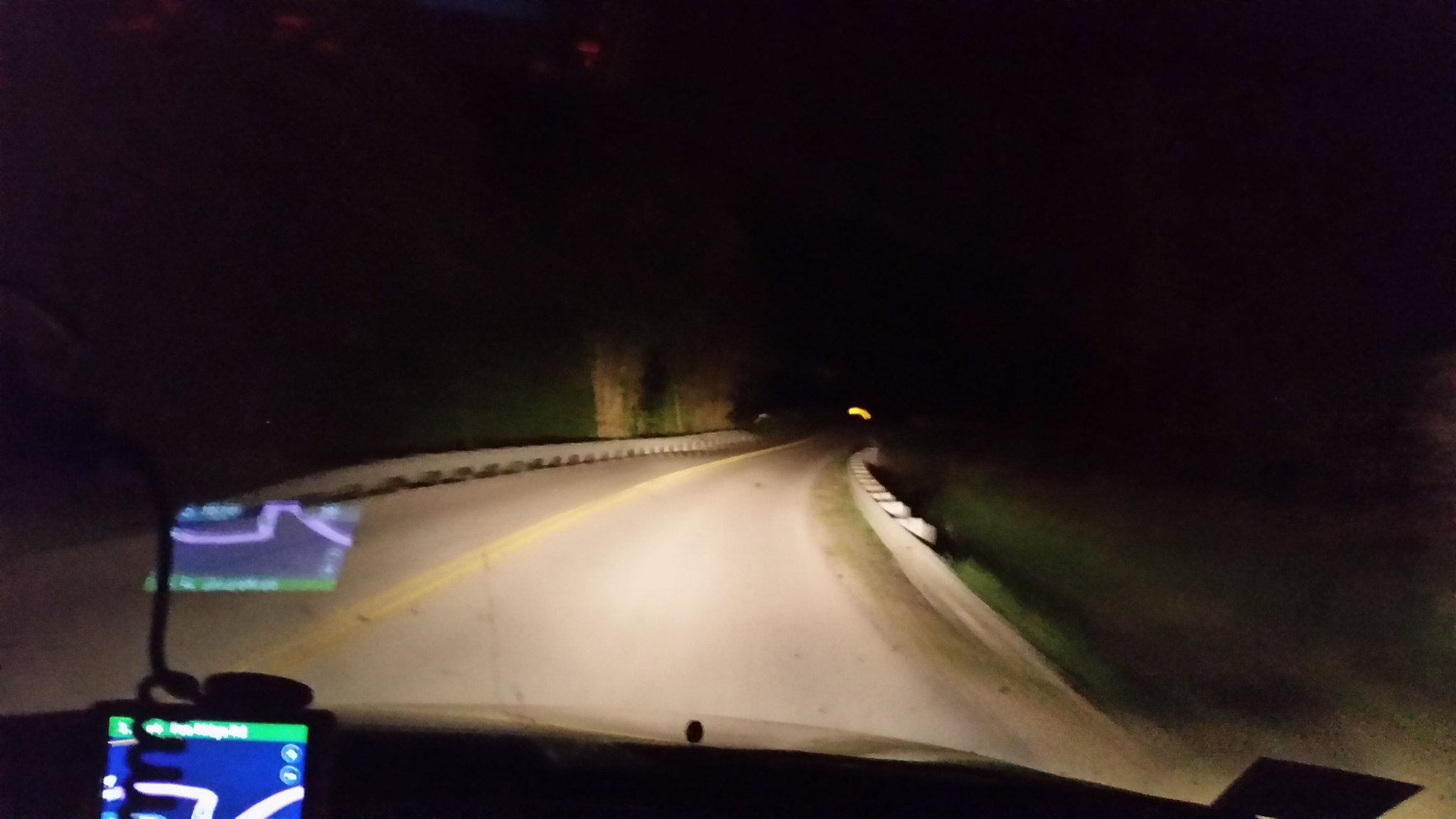In this nighttime photo taken from inside a moving car, the interior elements and the road ahead create a vivid scene. The car's front dashboard is partially visible, with a sticker decal adorning the bottom right side of the windshield. Mounted on the left bottom of the frame is a GPS device, connected by a spiral wire that curves upward. The GPS screen displays a green line across the top, transitioning to blue below, with a prominent white line indicating the route. The road itself is a two-lane passage, demarcated by metal guardrails on both sides. In the distance, a light signals the presence of either oncoming traffic or a vehicle further along the road. The right side of the roadway is edged with green vegetation, while trees rise behind the left-side guardrail, partially obscured by the night.